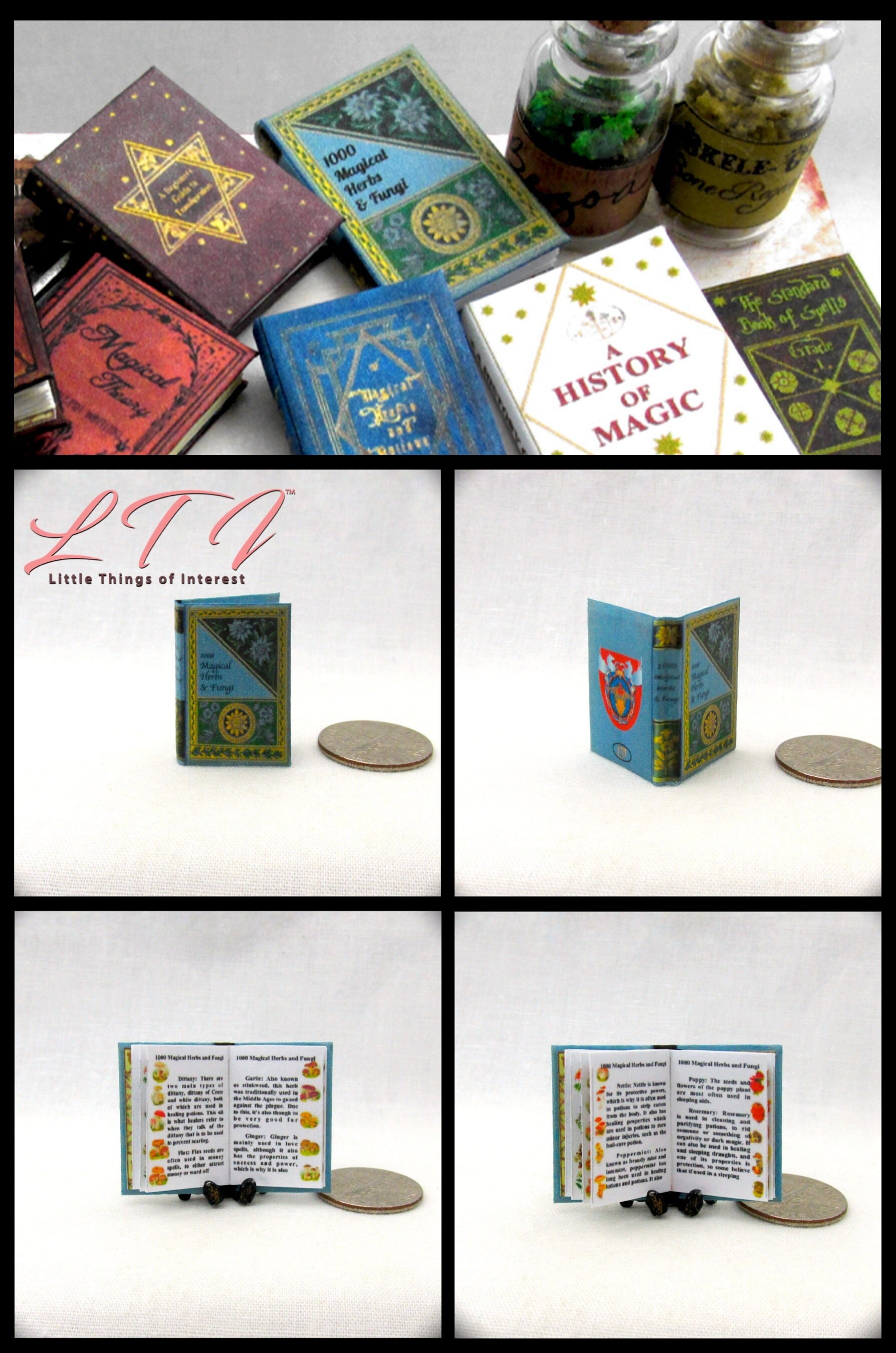This detailed image showcases a five-panel display of various magic-related books and jars. The top panel, which stretches across the full width of the display, presents five distinct books accompanied by two jars containing crystal-like substances. Among these books are titles such as "A History of Magic," "A Thousand Magical Herbs and Fungi," "Magical Theory," and "The Standard Book of Spells." The book "The Magical Herbs and Fungi" bears the text "LTI" in cursive above it and "Little Things of Interest" below it, with a shield-like emblem featuring two birds on the spine. The bottom section is divided into four equal-sized panels, each showcasing a detailed blue and green book against a white background. The first panel features the book closed and upright, the second displays the book open with pages facing away from the viewer, and the third and fourth show the book open with printed pages visible. A small coin next to these books provides a scale, indicating the miniature size of these items. The arrangement and detailed presentation underscore the magical theme of the collection.